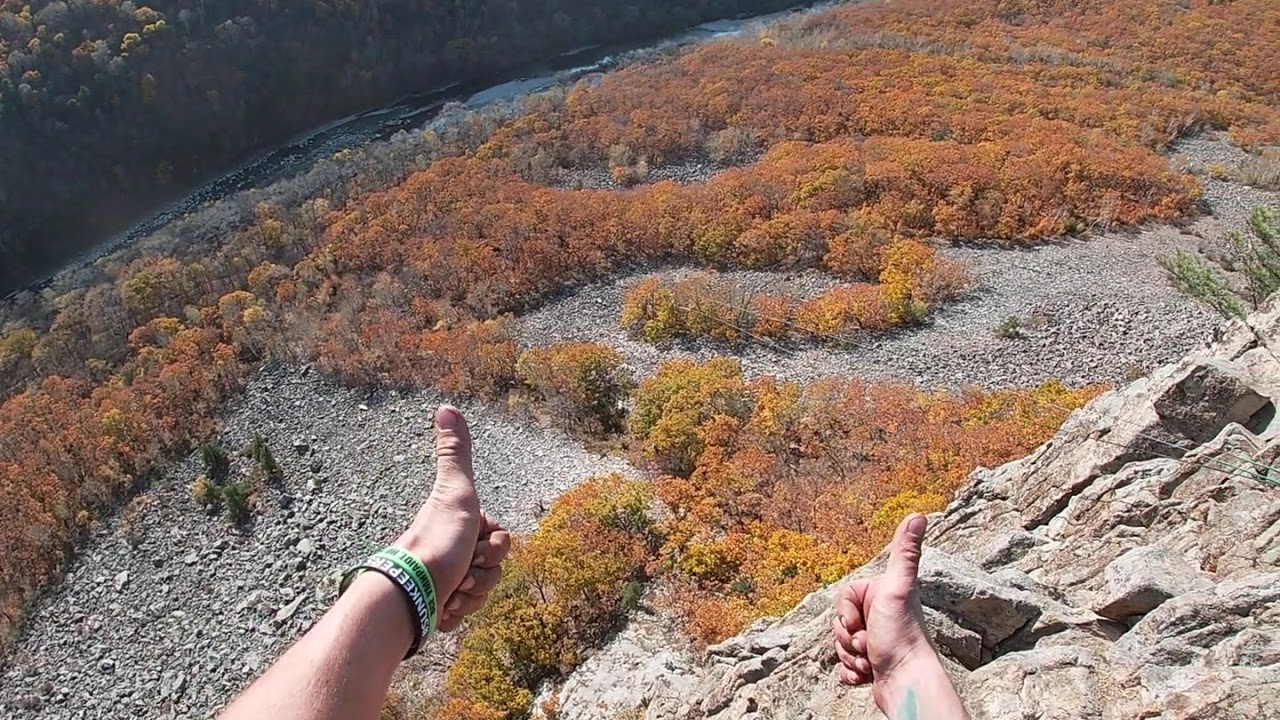The photograph captures a breathtaking autumn scene from the perspective of someone standing or sitting on the edge of a rocky cliff, likely shot using a GoPro mounted on their head. At the bottom of the frame, the person's hands, with white skin, are visible giving enthusiastic thumbs-up gestures. The left wrist is adorned with two bracelets. The rugged cliff is framed in the bottom right corner, emphasizing the steep drop-off below. The expansive landscape reveals a dense forest with vibrant fall foliage, predominantly orange, yellow, and red leaves. Among the sea of treetops, patches of exposed rocks and gravel are visible. In the far background, a winding river cuts through the forest, leading to a distant area filled with greener trees. The scene perfectly encapsulates a hiker's triumphant moment, celebrating nature's beauty from a high vantage point.